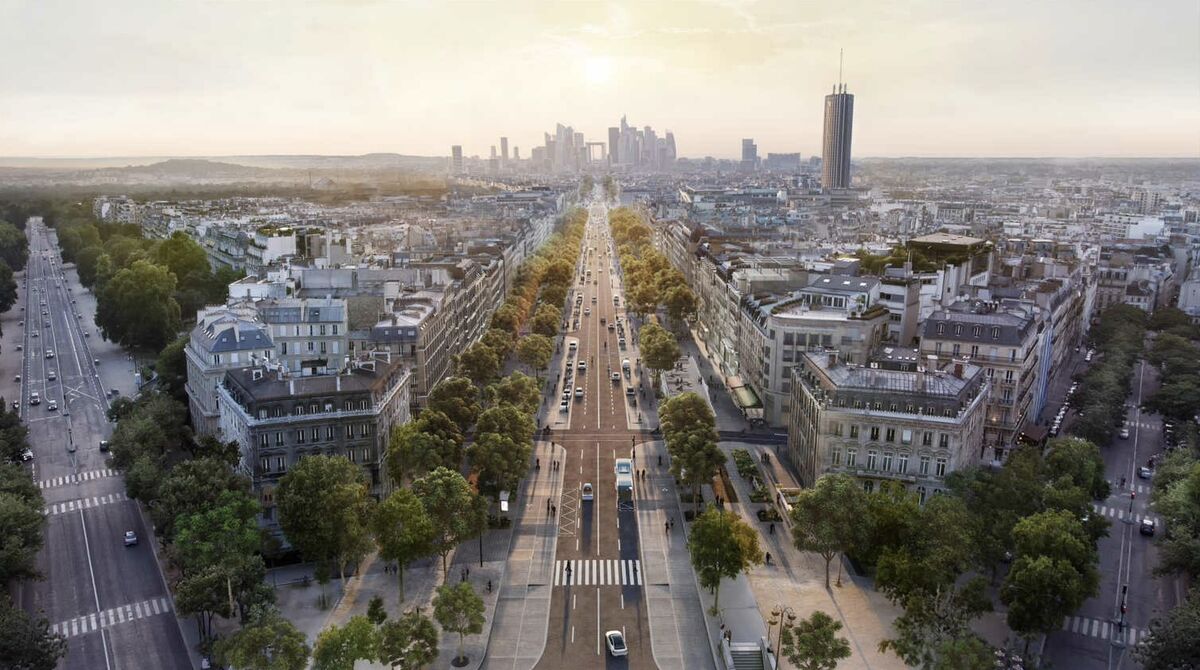This aerial view captures a sprawling cityscape marked by three prominent highways that converge toward a dense cluster of buildings in the distance, forming an almost V-shape. The central highway stretches straight from the foreground toward the city center, flanked on both sides by green trees. These trees line the highways and sidewalks, providing a stark contrast to the predominantly gray and beige structures. The left and right highways diverge from the central one, each lined with a similar arrangement of trees and buildings. The buildings between and alongside these highways are tall and closely packed, some appearing as residential apartments.

In the background, the city's skyline is dominated by large skyscrapers and a distinctive bridge with a square arch. The overcast sky casts a gray hue over the entire scene, blending with the grays of the buildings, roads, and horizon. The sun sits directly above, partially obscured by the clouds, offering a muted light over the cityscape. The image conveys a sense of depth and distance, stretching from the densely structured outskirts to the towering high-rises at the core, framed by a mix of bustling highways and verdant trees.